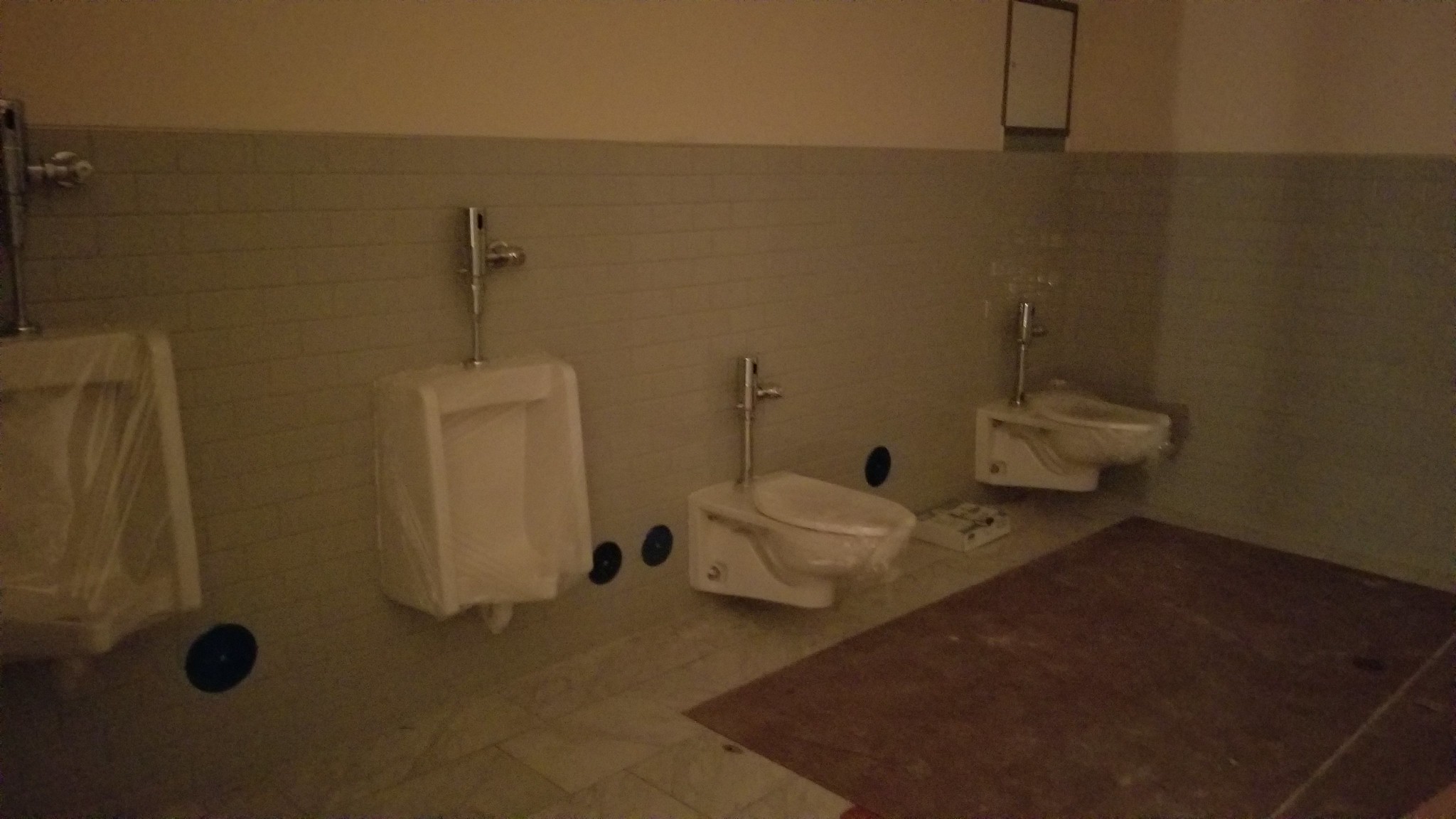This photograph captures a dimly lit, slightly blurry image of an unfinished men's restroom under construction. The walls are tiled with pale green subway tiles that extend about halfway up, transitioning to a white color above. The floor consists of mismatched tiles, with sections of white marble and dark brown or light maroon tiles, suggesting repairs or incomplete installation.

On the back wall, there are two urinals to the left and two wall-mounted toilets to the right, all wrapped in clear plastic, indicating they have just been installed. The absence of stalls or dividing walls between the fixtures suggests that the construction is not yet complete. Silver pipes are visible above the fixtures, and four black circles can be seen towards the bottom of the wall, possibly placeholders for future installations or fittings.

A small rectangular opening is present on the right edge of the room, and there is a feature above the last toilet that might be a mirror or a small cabinet. The ambient lighting is dim and grainy, with no apparent lighting fixtures turned on, further emphasizing the ongoing construction status of the bathroom.